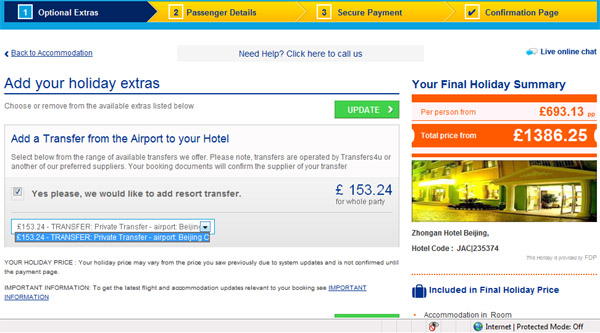**Holiday Package Overview: Optional Extras, Passenger Details, and Secure Payment Process**

---

At the top left of the page, the header reads "Optional Extras" in blue, accompanied by a number "1". The subsequent sections are highlighted in yellow:

1. **Passenger Details:** Indicated by the number "2".
2. **Secure Payment:** Indicated by the number "3".
3. **Confirmation Page:** Indicated by a checkmark, signifying the completion of the process.

Below these sections, the main body of the page begins. The top left features a link titled "Back to Accommodation" and another link stating "Need help? Click here to call us" followed by "Live Online Chat".

Highlighted in blue text is the option to "Add Your Holiday Extras", directly followed by instructions to "Choose to remove from the available extras listed below". 

An option to "Add a transfer from your airport to your hotel" is presented. There’s a prompt to "Select from the range of available transfers we offer". Important information is given about the transfer service:

- Transfers are provided by "Transfers for you" or another preferred supplier.
- Booking documents will confirm the exact transfer supplier.

A checkbox is available to opt-in with the text: "Yes please, we would like to add a resort transfer". The cost for this service is listed at £153.24 for the whole party, displayed in a separate small box specifying "£153.24 Private Transfer, Airport to Beijing Hotel".

On the right side of the page, there is an image of a hotel. Below the image, the "Final Holiday Summary" is detailed:

- **Per Person:** £693.13
- **Total Price:** £1,386.25 for the entire 3-night stay.